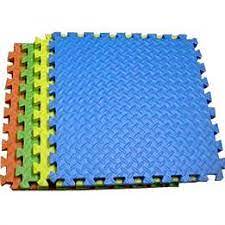This image is a high-quality product photograph likely intended for an Amazon listing. Featured are four interlocking floor mats, each with a distinct color and puzzle-piece-like edges that allow them to connect seamlessly. The mats, which appear cushioned and textured for added comfort, are stacked in a visually appealing manner to showcase both their full design and color options. At the top of the stack is a blue mat, followed by a yellow mat, a green mat, and a red mat. These mats are typically used in environments like preschools, kindergarten classrooms, or gyms, offering a versatile solution for creating safe play areas or cushioned workout spaces.